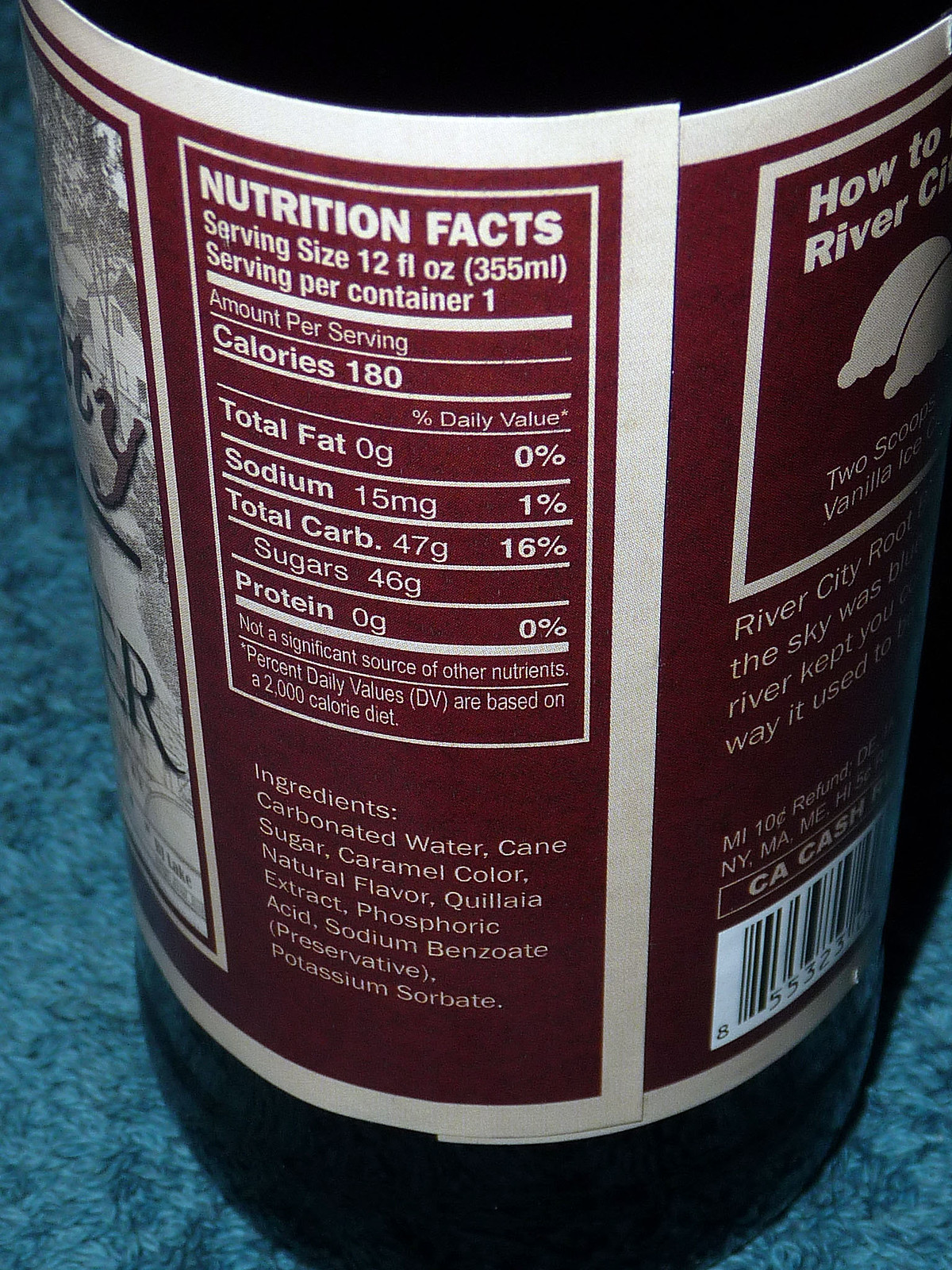This close-up photograph showcases a bottle filled with a dark liquid, resembling Coca-Cola or a similar type of carbonated drink, placed on a light blue or teal surface. The bottle is adorned with a maroon label featuring white text and borders, prominently displaying Nutrition Facts. The label details include a serving size of 12 fluid ounces (355 milliliters) with 180 calories per serving, zero fat, 15 milligrams of sodium, 47 grams of total carbohydrates, 46 grams of sugar, and zero grams of protein. The ingredient list at the bottom mentions carbonated water, cane sugar, caramel color, natural flavor, quillaja extract, phosphoric acid, sodium benzoate, and potassium sorbate. On the left side of the label, a partial image reveals a pathway leading to a house with trees, whereas the text on the right side includes partial words ending in "T-Y" and "E-R," a brand description, and a barcode. The bottle itself appears to have a dark brown or black tint.